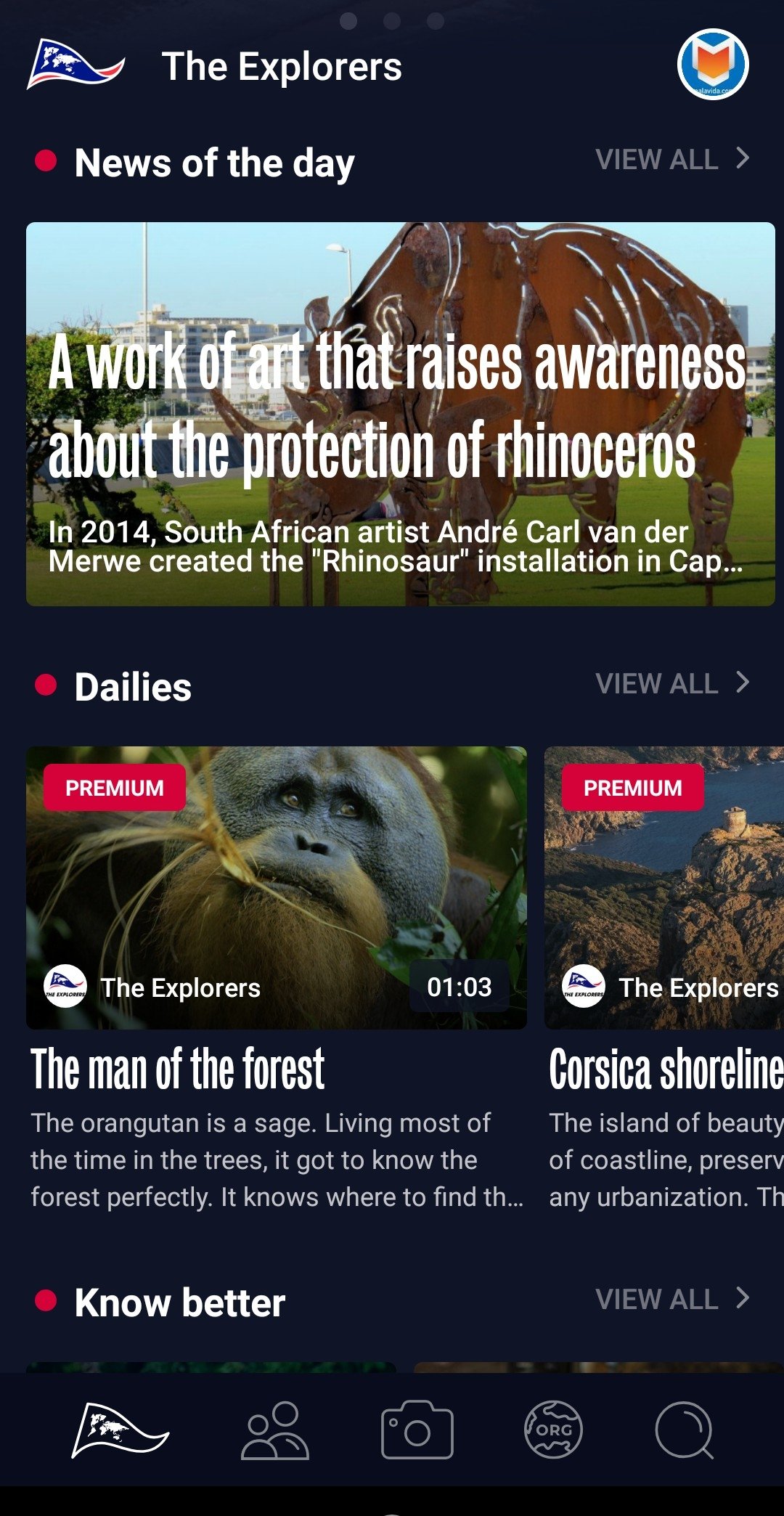The image titled "The Explorers" is showcased on a "News of the Day" page. The title, "The Explorers," is prominently displayed in white font on the upper left-hand side against a black background. Adjacent to the title is an icon resembling a flag—a bluish banner with a red tip. On the upper right-hand side, there is a circular emblem featuring a white edge and a blue middle, containing a silhouette that resembles an "M" with an orange object underneath, giving the impression of a face or head.

Below this emblem, the words "News of the Day" are displayed, leading to a wide square nearly spanning the width of the image. This square contains the message, "A work of art that raises awareness about the protection of rhinoceros," written in white font centered on the image. Behind this text, a rhinoceros is depicted, with what appears to be a business building in the background.